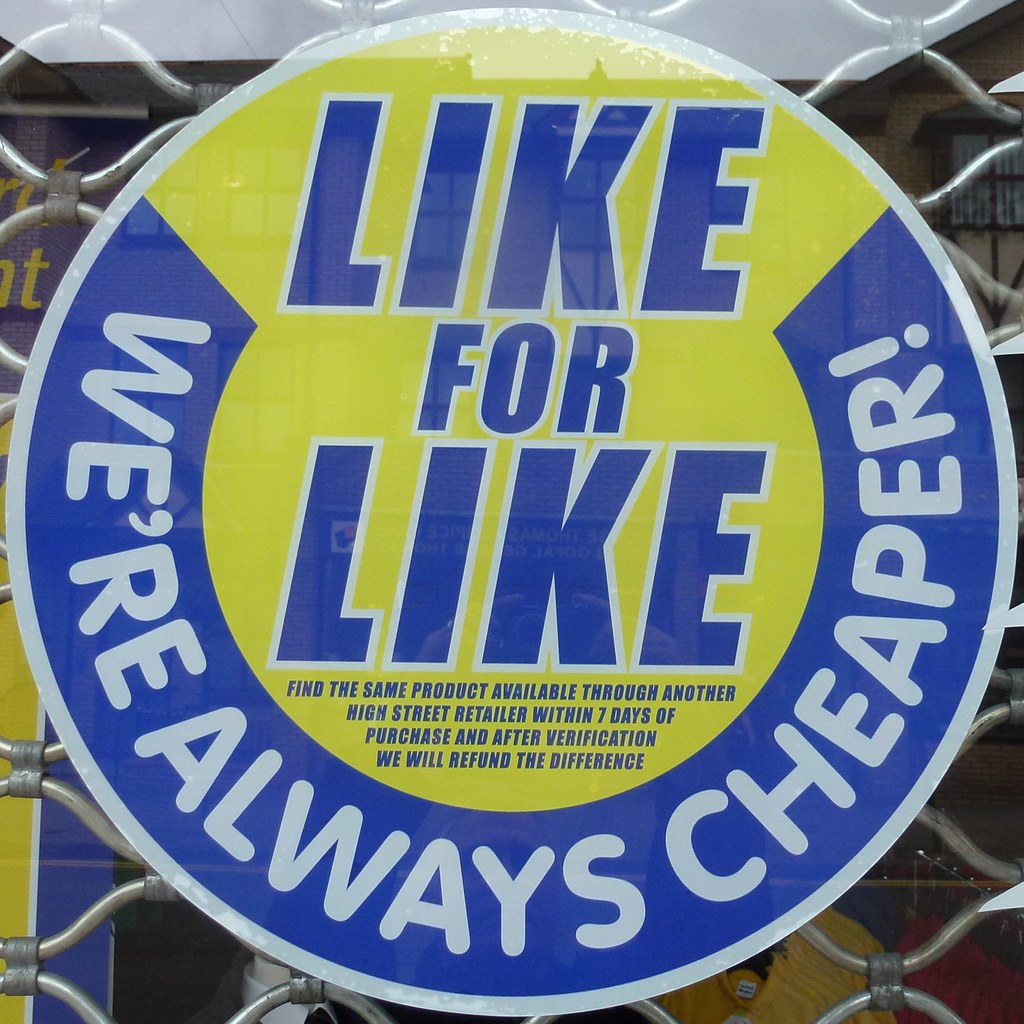The image shows a circular ad decal attached to a window, with reflections indicating it's positioned against decorative steel fencing. The center of the circle is bright yellow with the bold blue capitalized text, "LIKE FOR LIKE." In smaller blue text beneath, the ad explains: "Find the same product available through another high street retailer within 7 days of purchase, and after verification, we will refund the difference." A blue semicircle at the bottom of the ad features white text in a casual, almost comic sans font, stating: "WE'RE ALWAYS CHEAPER!"